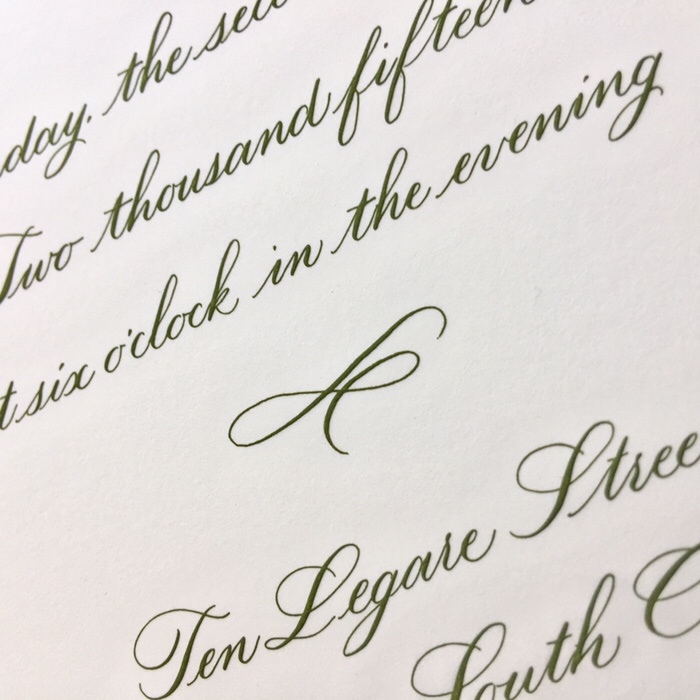This close-up photograph captures cursive text on a creamy white paper with a slightly grayish tinge. The text, appearing dark gray verging on black with a faint greenish hue, is at a 45-degree angle relative to the viewer. The visible first line consists of the partially cut-off words "day, the, se." Below that, the text reads "2015" followed by "six o'clock in the evening." Centrally located beneath this is an abstract swirled pattern in the same dark color. Further down, the text, again partially cut off, read "10 Laguerre Street," followed by the partially visible word "south" at the bottom. The intricately written cursive text and formal layout suggest that this could be part of a wedding invitation or a special event announcement. The edges of the paper are not fully visible, cutting off various portions of the text, making it an incomplete, yet elegant snapshot.